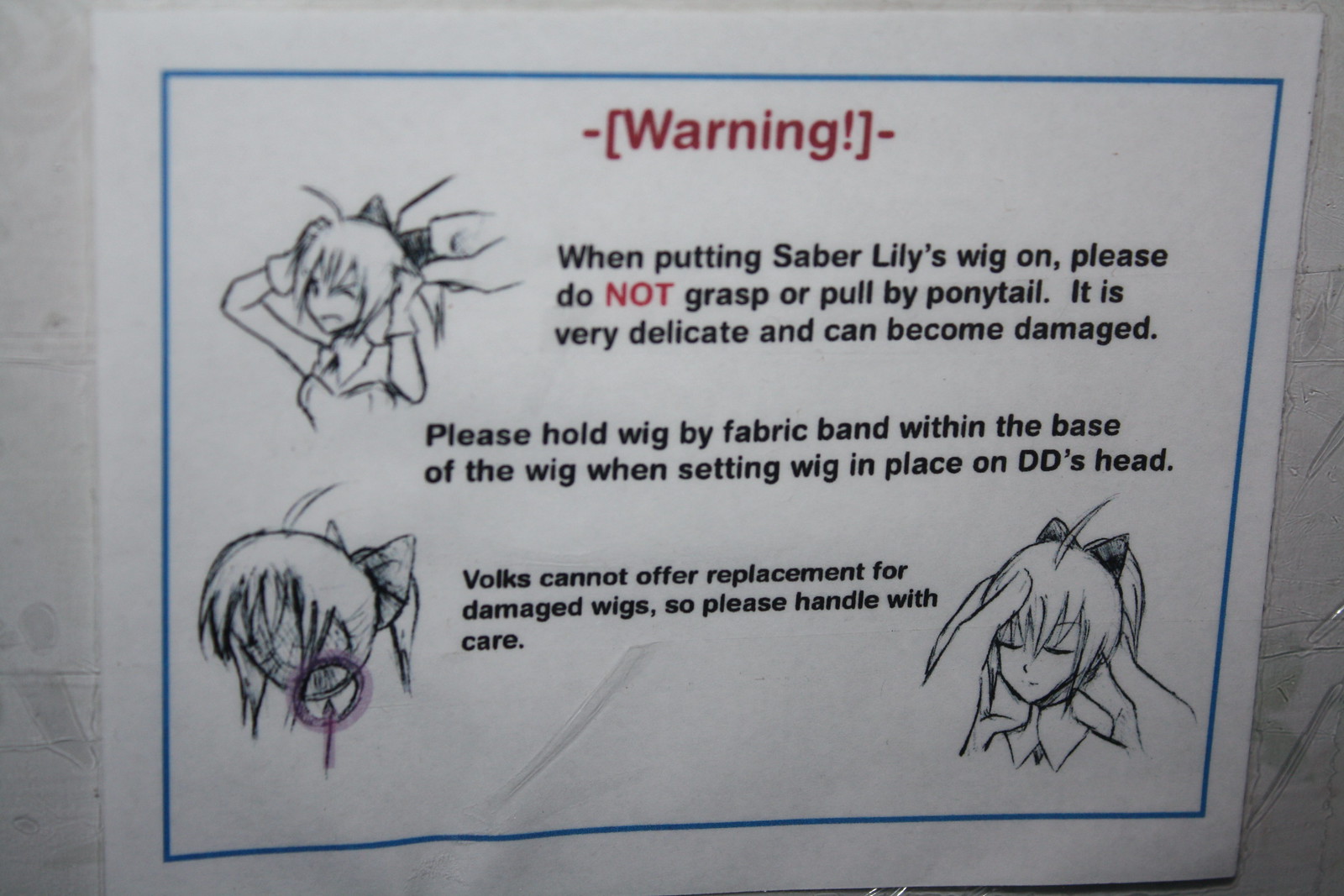The image shows a warning poster taped on a door. The poster is a plain piece of white paper with a blue border. At the top of the paper, the word "WARNING!" is written in red, enclosed in brackets, and flanked by two small lines on each side. Below this, the text reads: "When putting Saber Lily's wig on, please do NOT grasp or pull by the ponytail. It is very delicate and can become damaged." The word "NOT" is in uppercase and also red. Further instructions state: "Please hold the wig by the fabric band within the base of the wig when setting the wig in place on Didi's head." Another caution follows: "Vox cannot offer replacements for damaged wigs, so please handle with care." Surrounding the text are pictorial guides, including sketches of an anime-style girl. On the left, an image depicts someone pulling a ponytail and a woman frowning. To the right, there is another image of a woman calmly smiling as she places the wig on a doll’s head, illustrating the correct method.